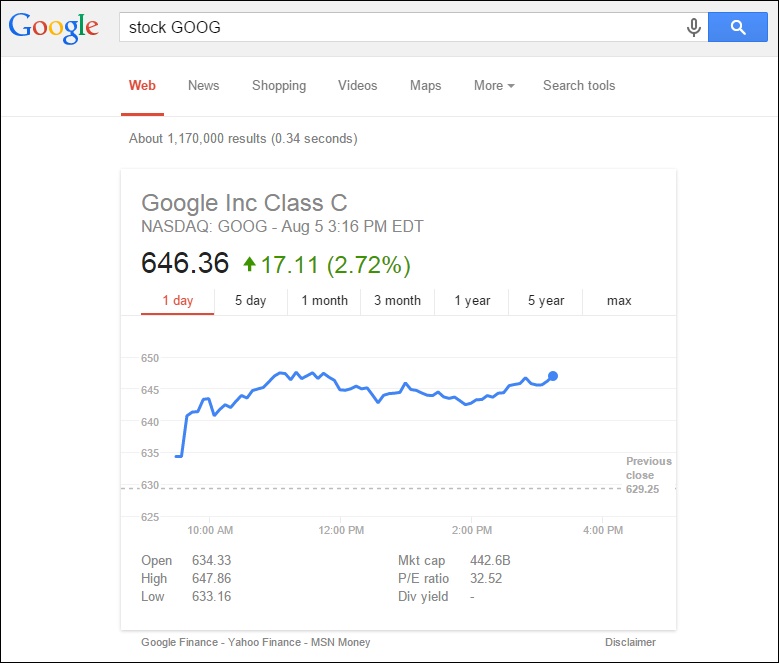Here is a cleaned-up and detailed caption for the image described:

---

This screenshot captures a detailed view of a stock market analytics page, specifically focused on Google's stock (GOOG). At the top, the Google icon is prominently displayed beside a search bar, which contains the text "GOOG" indicating a search for Google's stock information. The search bar also features a microphone icon for voice search and ends with a blue search button. Below the search bar, a series of tabs are visible, including options for Web, News, Shopping, Videos, Maps, and More. The tab labeled "Web" is highlighted in red.

Under this tab layout, the page indicates approximately 1,170,000 results fetched in 0.34 seconds. The subsequent section presents the stock's information: "Google INC Class C" is written in large gray letters, followed by "Nasdaq: GOOG – August 5, 3:16 PM EDT" in smaller gray print. The current stock price is displayed prominently in large numbers as $646.36, alongside a green upward arrow indicating a rise of $17.11 (2.72%).

Further down, the screenshot includes a line chart illustrating the stock's performance. The blue line on the chart starts slightly below $635 (approximately $633) and concludes around $646. The chart's tabs offer various time frames for analysis, such as 1 Day, 5 Day, 1 Month, 3 Month, 1 Year, 5 Year, and Max, with additional opening and closing price details at the bottom.

---